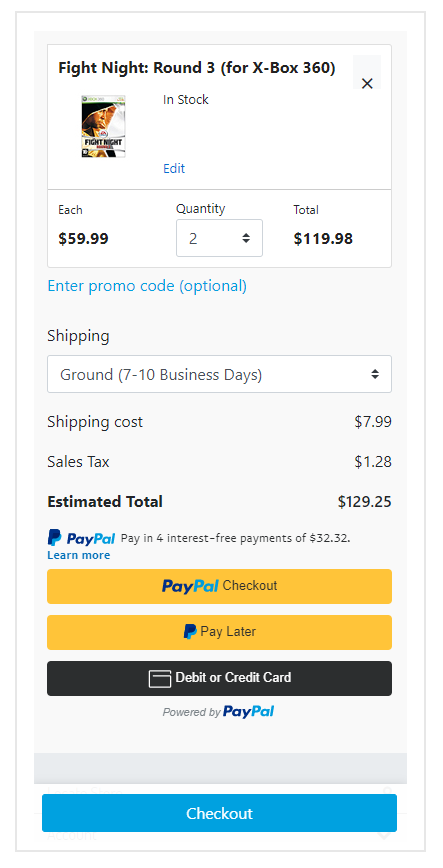The image displays the checkout page for the video game "Fight Night Round 3" for Xbox 360. At the top, there is a small image of the game's CD cover. The page indicates that each game is priced at $59.99, and two copies have been ordered for a total of $119.98. Underneath the game details, there's an "Edit" button, whose function isn't specified. 

The white background features a section where users can enter a promo code, which is optional. Shipping is set to Ground, taking 7-10 business days, with a shipping cost of $7.99. Sales tax adds an additional $1.28, bringing the estimated total to $129.25. 

Below these details, three payment options are displayed prominently:
1. **PayPal** - Offering interest-free payments of $32.32.
2. **PayPal Checkout** - A standard checkout option via PayPal.
3. **PayPal Pay Later** - Allowing users to pay at a later date.

There is also a dark button option for paying with a debit or credit card, powered by PayPal. At the bottom of the page, there's a prominent blue "Checkout" button, finalizing the purchase process.